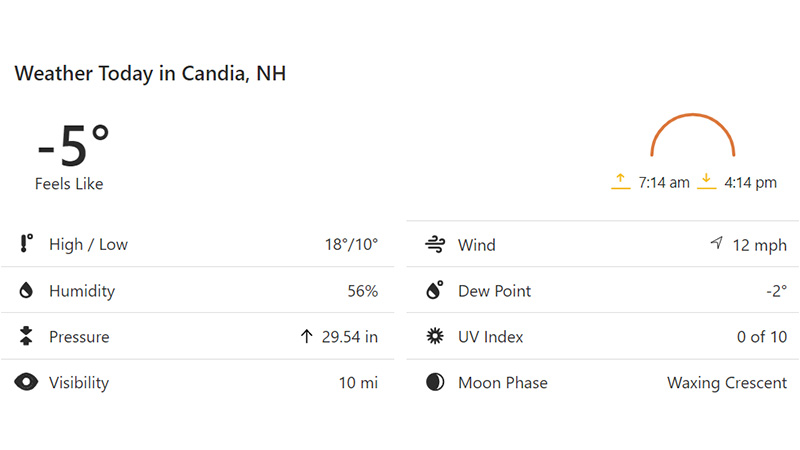This detailed weather forecast screenshot for Candia, NH features a clean, white background with "WEATHER TODAY IN CANDIA, NH" prominently displayed in black in the top-left corner. Below this title, the temperature is shown as -5 degrees, with "feels like" indicated in a smaller font beneath it.

To the right of this information, there is a red half-circle graphic. On the left side of the half-circle, there is an upward-pointing arrow alongside "7:14 a.m." signifying the sunrise time. On the opposite side, a downward-pointing arrow is next to "4:14 p.m.," marking the sunset time.

Below these primary details, there are two distinct columns each containing four rows:

**Left Column:**
1. A thermometer icon indicates the high/low temperatures as 18°F/10°F.
2. A water drop symbol shows the humidity at 56%.
3. Two arrows pointing at each other denote pressure, with an up arrow indicating 29.54 inches.
4. An eyeball icon signifies visibility, recorded at 10 miles.

**Right Column:**
1. A wind symbol describes the wind direction with an arrow and lists the wind speed at 12 miles per hour.
2. A water drop with a small dot next to it notes the dew point at -2°F.
3. A sun icon indicates the UV index being 0 out of 10.
4. A circular icon with a sliver of white, resembling a crescent moon, informs about the moon phase, stated as waxing crescent.